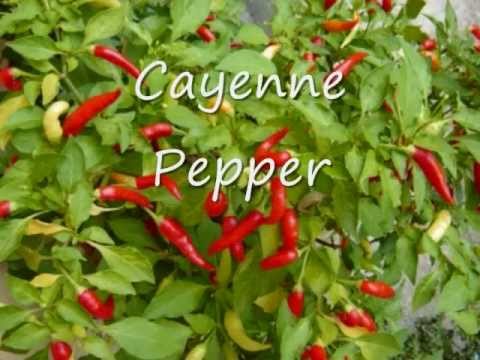The image portrays a close-up view of a vibrant garden scene featuring numerous bright red cayenne peppers. The peppers, long and pointed with a shiny surface, are interspersed among predominantly light green leaves, some of which have jagged edges and yellowish hues. A few underdeveloped green peppers are also visible, indicating various stages of ripeness. Central to the composition, in slightly off-centered white text, are the words "cayenne pepper." The background reveals subtle patches of gray, suggesting an outdoor setting with a sky-like or natural backdrop. The overall aesthetic of the image resembles a detailed painting or drawing, capturing the lively essence of the garden.